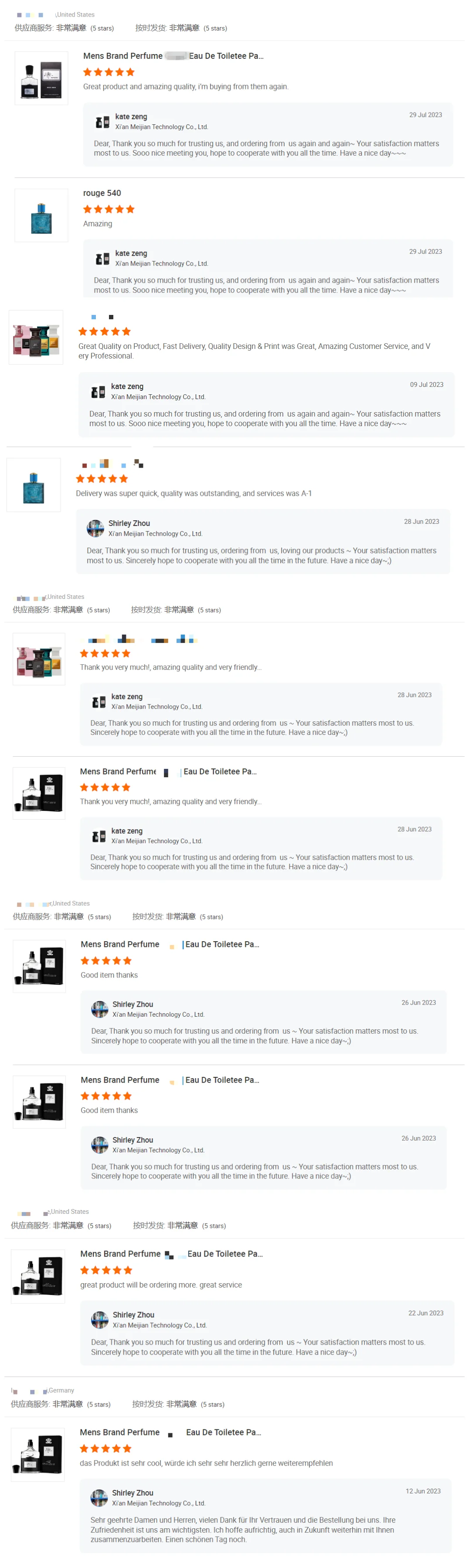This image features a neatly organized grid of 11 items, each comprising a small, detailed picture on the left and a descriptive text on the right. The overall image quality is low, making it somewhat difficult to read the finer details. Each item includes a title at the top in bold black font, followed by a brief description in a lighter gray font. Directly below the description, there are star ratings and a summary of user reviews, enclosed in a gray box. Several of these items appear to be men's perfumes, indicated by readable text on some of the images. Additionally, a few items feature text that looks like Chinese characters, suggesting a diverse range of products.